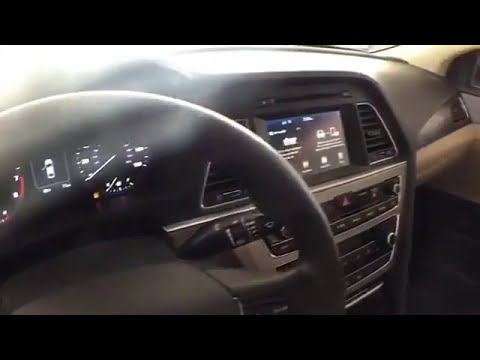This photograph captures the detailed interior of a modern vehicle, primarily focusing on the driver's side. The scene prominently features a black leather steering wheel and a lit speedometer, currently reading zero. The dash displays important indicators including the fuel gauge, which shows the car is on empty with the gas light illuminated in pale yellow. There's also an icon indicating the driver's door is open. Surrounding these indicators are various control knobs and buttons for adjusting the heater, air conditioning, and defrosters. The sleek dashboard, combining a grayish and black-and-silver color scheme, integrates seamlessly with a digital screen embedded in the center console, adding to the high-tech ambiance. No seats are visible in this shot, emphasizing the pristine, well-organized layout of the dashboard and driver’s side controls.